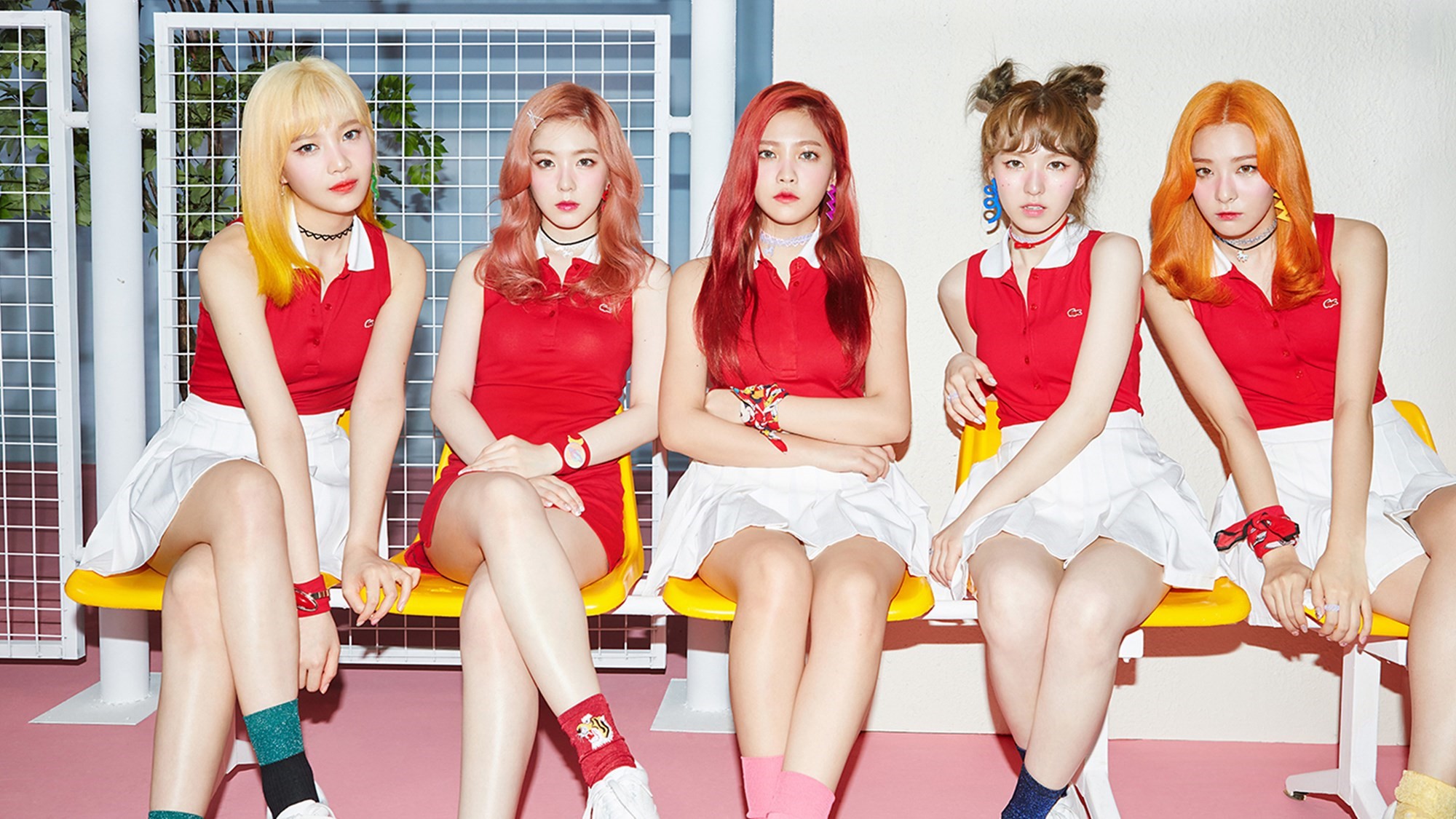The image depicts an indoor setting with a white wall in the background and a white net fence gate with metal poles on the left side. The floor is a distinct pink color. Five young women, likely of Asian descent and appearing to be members of a K-pop band, are seated on interconnected yellow plastic benches with white legs. They all sport eye-catching, multicolored hair, which includes shades of blonde, maroon, brown, and bright orange, with various styles such as long hair, bangs, and buns. The women are uniformly dressed in a color scheme of red and white; each is wearing a red top and white skirt, consistent with an outfit reminiscent of tennis attire. They sit in a row, looking serious and composed, adding to the stylish and vibrant atmosphere of the scene.